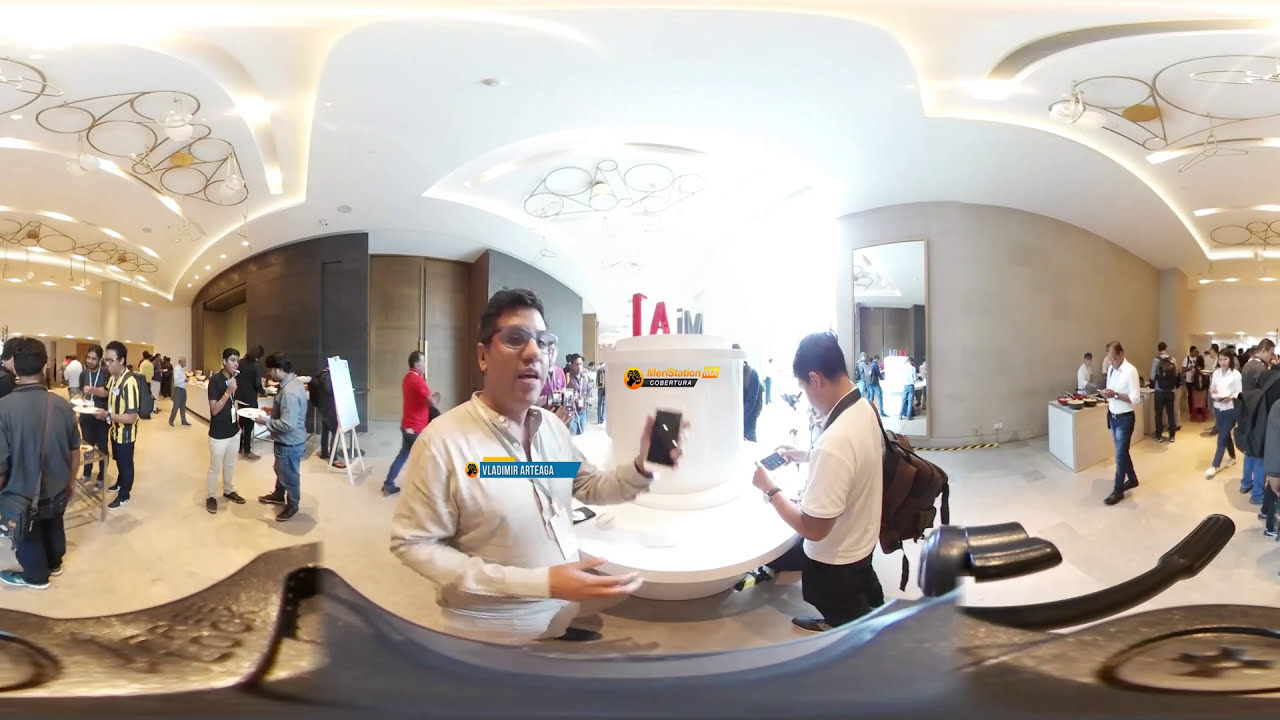The image captures a vibrant and bustling convention or conference set in what appears to be a hotel lobby or convention center. The panoramic, 360-degree view showcases an expansive, open room adorned with a bright white ceiling featuring decorative circular metal designs, some resembling bicycle frames. The fisheye lens distorts the scene slightly, bringing some elements closer and pushing others farther away.

At the center of the image is a man prominently featured with medium skin, black hair, glasses, and a white long-sleeved shirt. He holds a smartphone with a white body and black screen high in his left hand, while his right hand is mid-gesture, possibly indicating he is speaking. Above him is a blue banner with white text that reads "Vladimir Ortega," accompanied by a logo. Near him, to the right, stands another man in a white short-sleeved polo shirt, focusing intently on his own phone held horizontally and sporting a backpack on one shoulder.

The scene is lively with many groups of people milling about, all wearing lanyards, suggesting an organized event. Stands and tables are set up throughout the room, with some attendees holding plates of food. The floor is tiled, and light floods the space from a bright, natural source at the top center of the image. Large, tall doors framed by a wood-effect brown wall in the background contribute to the open and welcoming feel of the lobby area. The image captures a rich tapestry of interactions and engagements typical of a bustling convention atmosphere.